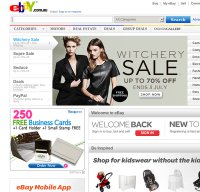This screenshot appears to be from an older eBay webpage, likely dating back to the early to mid-2010s. The page features a prominent advertisement for a sale, with the tagline "For Sure Resale," showcasing two women dressed in black. The sale boasts up to 70% off and is marked for July 3rd. Additionally, there is a "Welcome Back Sale" banner visible.

One distinct offer displayed is a promotional deal providing 250 free business cards, one card holder, and one small stamp at no cost. These items are depicted in the image.

The page includes a menu that presumably lists other sales and services, but the text is blurred and unclear even when zoomed in. The overall vintage aesthetic of the webpage, along with the type of advertisements and offers presented, suggests it's no longer a current eBay service model.